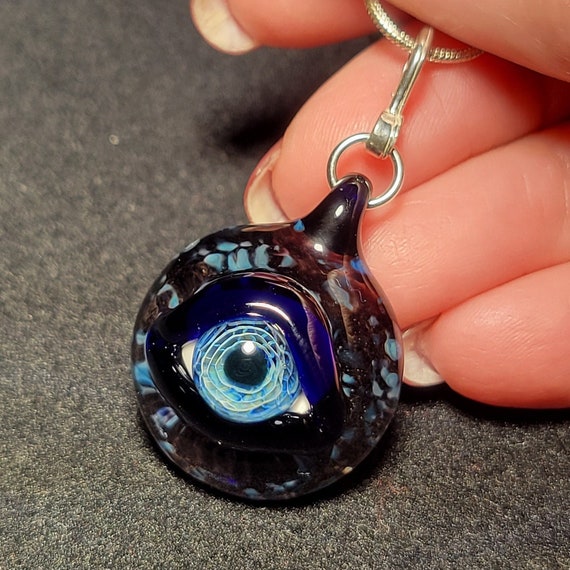The photograph features a woman with long fingernails holding an intricate circular glass pendant, roughly the size of two or three fingers wide. The pendant, which appears to depict an eyeball, has a strikingly glossy and shiny finish, with colors ranging from black and blue to hints of purple and white. The pendant is equipped with a small loop at the top for attachment, possibly making it part of a necklace or keychain. The setting is a gray, mottled background, and the woman's nails are painted, showing pink and white inside. She is holding the pendant delicately between her thumb and her pointer and middle fingers. The light reflects off the glass surface, emphasizing the vivid details of the eye within the pendant.